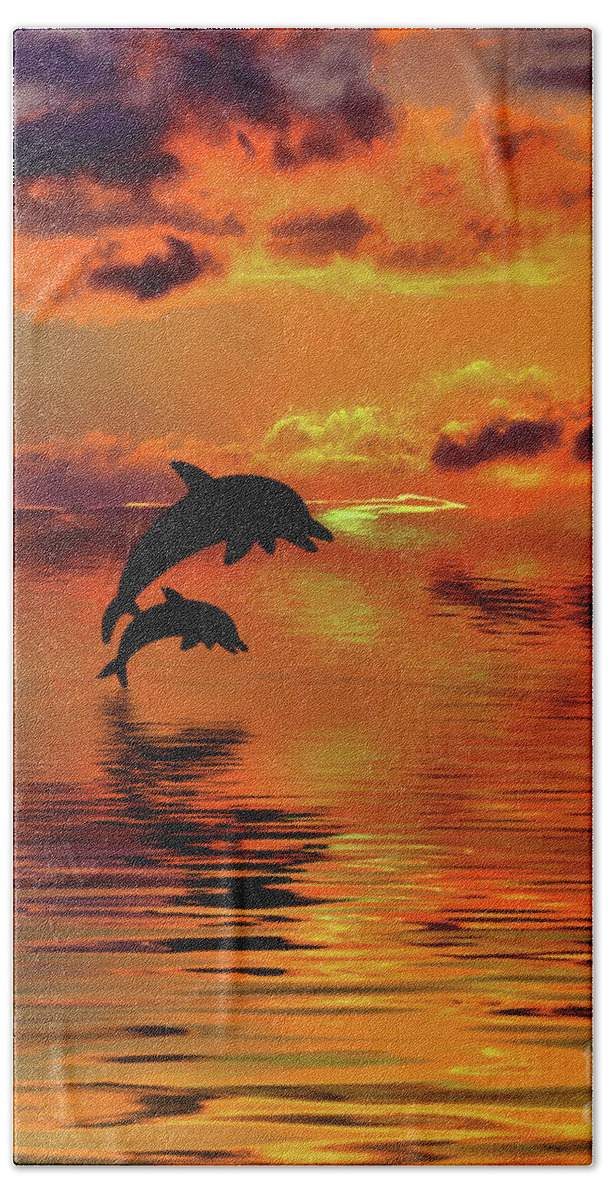This detailed image, resembling a painting, vividly captures an evocative scene of a sunset or sunrise over a large body of water. The vibrant palette of orange, yellow, and red dominates the entire scene, coloring both the sky and the water. Gentle ripples disturb the surface of the water, which is tinged with shades of orange and red from the setting or rising sun on the horizon. 

In the foreground, two dolphins are leaping out of the water, their forms silhouetted in black. The larger dolphin is positioned higher and further back, while the smaller dolphin is in the foreground, both casting shadows forward. The sky is filled with an array of clouds, predominantly orange, but transitioning to darker gray and even black towards the top and upper left-hand corner of the image. This masterful interplay of light and shadow enhances the overall magical and serene atmosphere of the scene, making it a striking representation of nature's beauty.